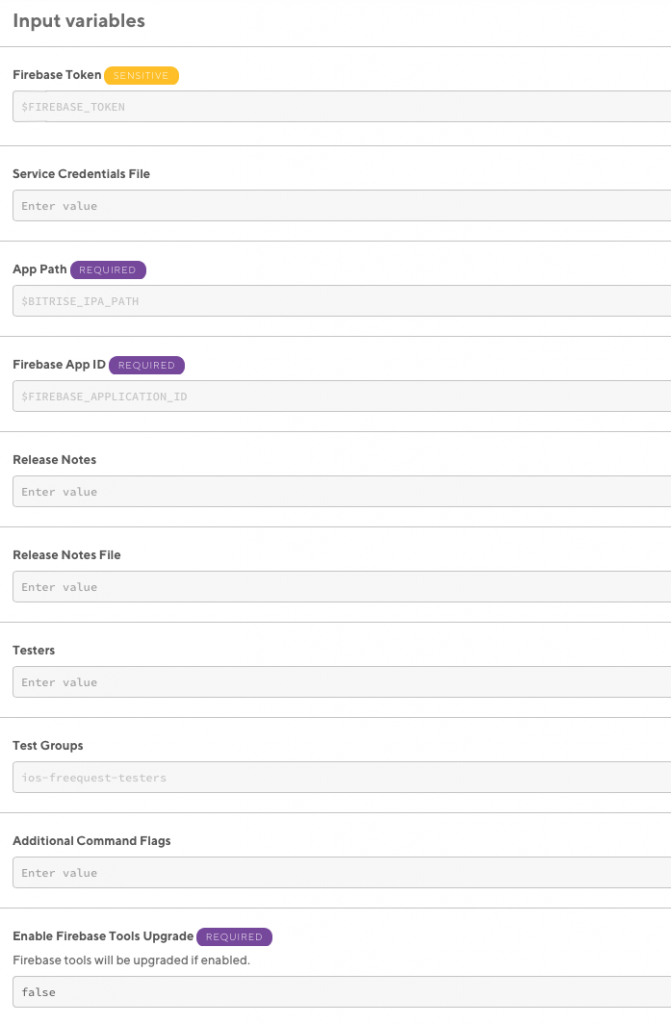At the top left, in bold gray lettering, the text "Input Variables" is prominently displayed. Directly beneath this heading, a thin gray line stretches across the entire page. Below this line, towards the left, "Firebase token" is written in bold black text. Adjacent to it, there is a yellow-orange filled oval containing faint white text that reads "Sensitive."

Underneath this section, there is an editable field framed by a medium gray border. Inside this field, the placeholder text reads "$FIREBASE_TOKEN" in all capital letters and gray font. This is followed by another horizontal gray divider. Further down the page, towards the left, "Service Credentials File" is labeled in bold black text. Below it, within a light gray background and framed by a gray border, is an editable area displaying the placeholder text "Enter value."

Another gray line acts as a separator before the next section. On the left, "Path" is written in bold black text, while on the right, a dark purple-filled oval with distinct spacing between white capital letters spells out "REQUIRED." Below this, an editable field showcases the placeholder text "$BITRISE_IPA_PATH" in all capital letters and gray font.

Continuing downward, a gray divider separates the next section. Towards the left, "Firebase App ID" is labeled in bold black text, and on the right, a similarly dark purple-filled oval contains white capital letters spelling out "REQUIRED." Below this, another editable field presents the placeholder text "$FIREBASE_APPLICATION_ID" in capital gray letters.

This detailed description encapsulates the layout and textual elements of the image, providing a clear and structured overview.